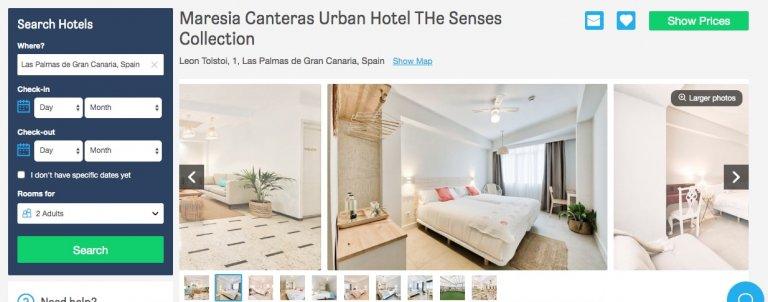**Caption:**

This screenshot from an unknown source displays a hotel search interface styled in a clean, user-friendly design. 

On the left, a search panel allows users to find hotels in "Las Palmas de Gran Canaria, Spain." It provides options to input check-in and check-out dates, select the number of rooms for two adults, and a checkbox for those without specific dates. Buttons labeled "Search" and "Need Help?" are also visible.

To the right, the featured hotel listing is for "Mauricia, Canteras Urban Hotel," located at "Leon Tolstoy I, Las Palmas de Gran Canaria, Spain." There is an option to show the map, along with icons for email and likes, and a prominent green button labeled "Show Prices."

Below the listing are three photos showcasing the hotel's interior. 

1. **Living Room:** The first image features a stylish living room decorated in cool white tones with a potted plant adding a touch of greenery.
   
2. **Bedroom:** The second image displays a cozy bedroom with a large bed, possibly formed by two smaller beds pushed together. The bed is dressed in white bedding with striking red throw pillows. Wooden nightstands flank the bed, and at the back of the room, there is a desk with a chair and another potted plant.

3. **Second Bedroom:** The final photo appears to be another bedroom featuring a white bed, a wooden desk accompanied by a white chair, and a comfy white armchair situated in the bottom left corner.

These images collectively highlight the modern, comfortable aesthetic of the Mauricia, Canteras Urban Hotel.